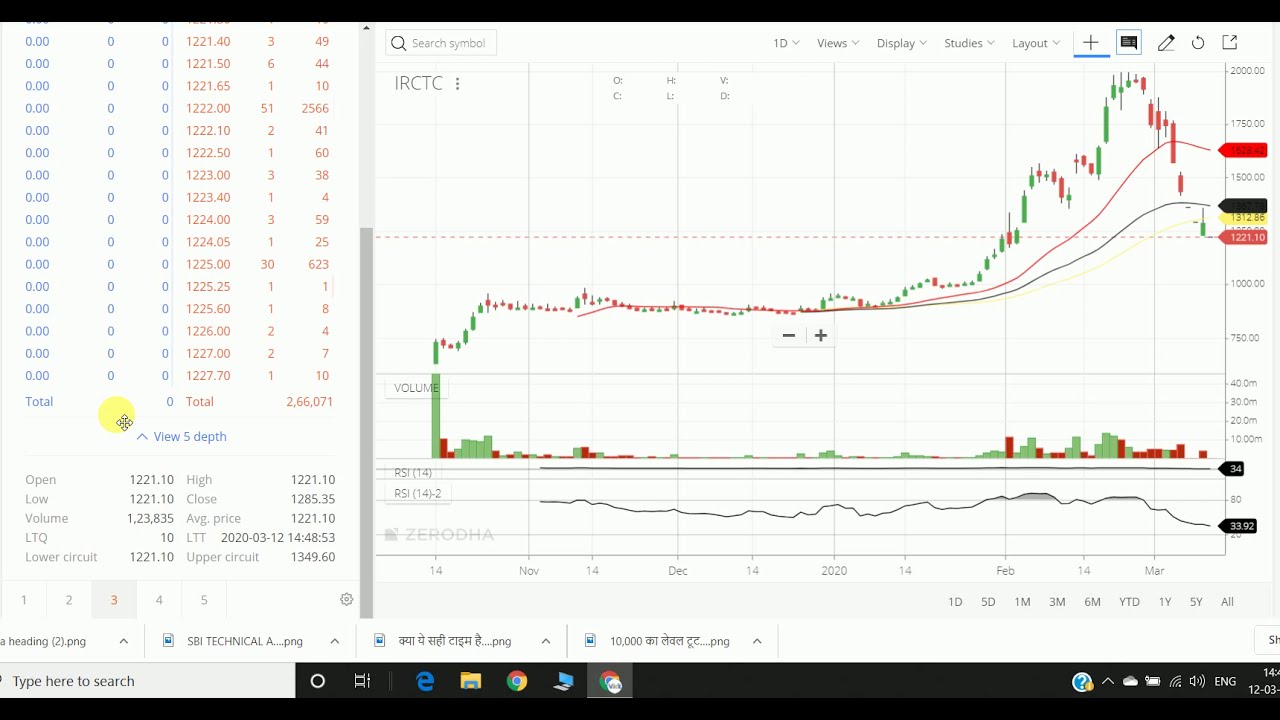The screenshot showcases a computer screen displaying a detailed stock trading chart for IRCTC. The user interface is characteristic of a Windows operating system, evidenced by the taskbar at the bottom. On the bottom left, the taskbar includes a 'Type here to search' field, along with icons for Edge browser, File Explorer, and Google Chrome, while the bottom right displays system icons for Wi-Fi, volume control, and partially cut-off time and date.

The primary focus of the screen is a trading chart from a program, possibly presented by a company called Zerodha. The chart is dated from 2020 and is visually vibrant with red and green colors illustrating the stock's performance metrics, including the open number, low number, volume traded, high of the day, closing number, average price, lower circuit, and upper circuit. The right-hand side of the chart features positive numbers at the top and negative numbers at the bottom, suggesting a baseline that moves upward. The left-hand vertical axis displays a range of values from zero up to the 1200s, indicating different stock prices or volumes. The chart aims to illustrate and possibly predict the stock's price movements, depicting the stock's fluctuations and market behavior over time. The image is well-lit, capturing the interface clearly and providing a comprehensive view of the details presented.